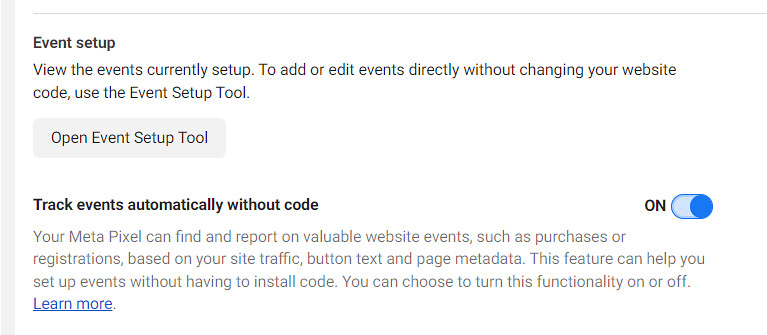### Detailed Caption

The image features a white background with a section on the top left labeled "Event Setup." Below this, there's a subheading that reads, "View the events currently set up to add or edit events directly without changing your website's code using the Event Setup Tool."

Under this heading, an option labeled "Open Event Setup Tools" is visible. Further down, there is a feature titled "Track Event Automatically Without Code." To the far right of this feature, there is an "On" switch displayed as a dark blue oval pill toggle, indicating that the feature is activated.

The description next to the toggle explains: "Your MetaPixel can automatically detect and report significant website events such as purchases or registrations based on site traffic, button text, and page metadata. This functionality allows you to set up events without having to install additional code. You can choose to turn this feature on or off." There is also a prompt to "Learn More" about the feature.